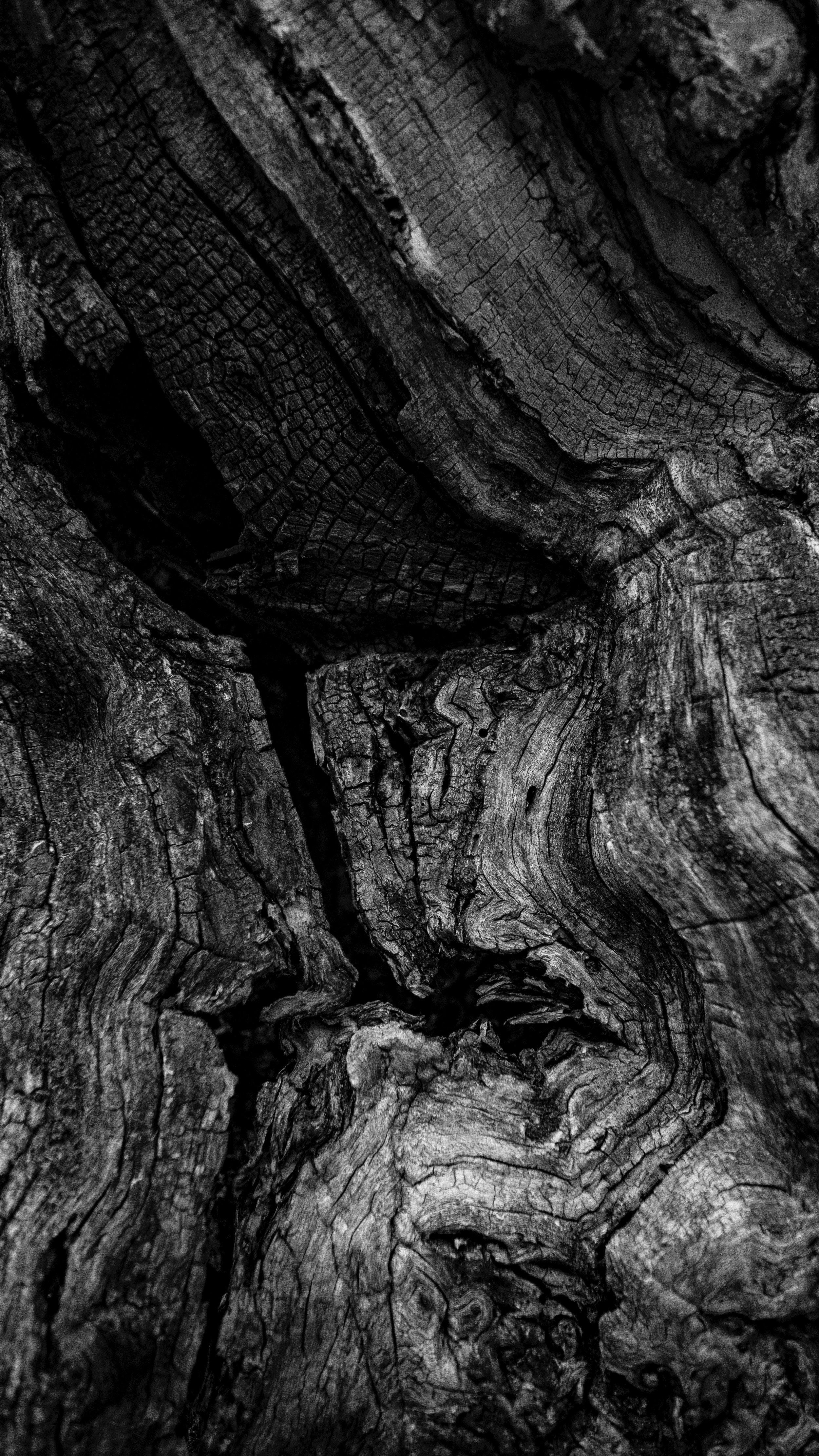The image is a black and white close-up photograph of a tree trunk with the bark mostly removed, revealing a highly textured and craggy surface. The portrait-oriented picture highlights a variety of intricate details, including a prominent knot in the lower middle section and another large knot with a significant opening. The top left portion resembles alligator skin with looping and curling grain patterns. The photograph features deep grooves and numerous cracks, some of which may be the result of charring or burning, as suggested by the contrasting shades of deep black, ash gray, and darker gray across the textured surface. These crevices and cavities enhance the gnarly and striking appearance of the tree trunk, making the image rich in detail and visually captivating.